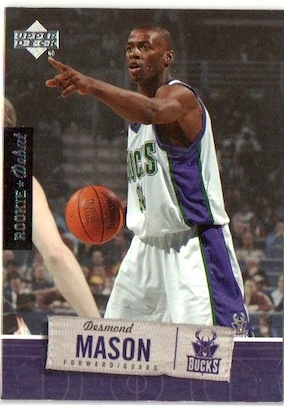This image features a basketball card in the upper left-hand corner, prominently displaying a dynamic shot of Desmond Mason, a player for the Milwaukee Bucks. He is wearing a white jersey with a blue stripe down the side and the word "Bucks" visible on it, though his number is obscured. Desmond Mason, who appears young with short hair, is depicted in action, dribbling the basketball with his right hand while his left arm is outstretched, pointing as if directing a play. To the left of him, there is a partial view of a defender, with just an arm and a bit of their head visible. The upper left corner of the card also features an emblem and some text, likely indicating the card company, though it's difficult to discern. On the left side, running vertically, there is a black rectangle with the word "Rookie" and Desmond's name. The lower section of the card includes a gray rectangular banner displaying "Desmond Mason" and his position "Forward/Guard", alongside the Milwaukee Bucks logo. The bottom portion of the card is shaded purplish, complementing the team's colors. The background of the main image includes spectators, suggesting a gym setting.